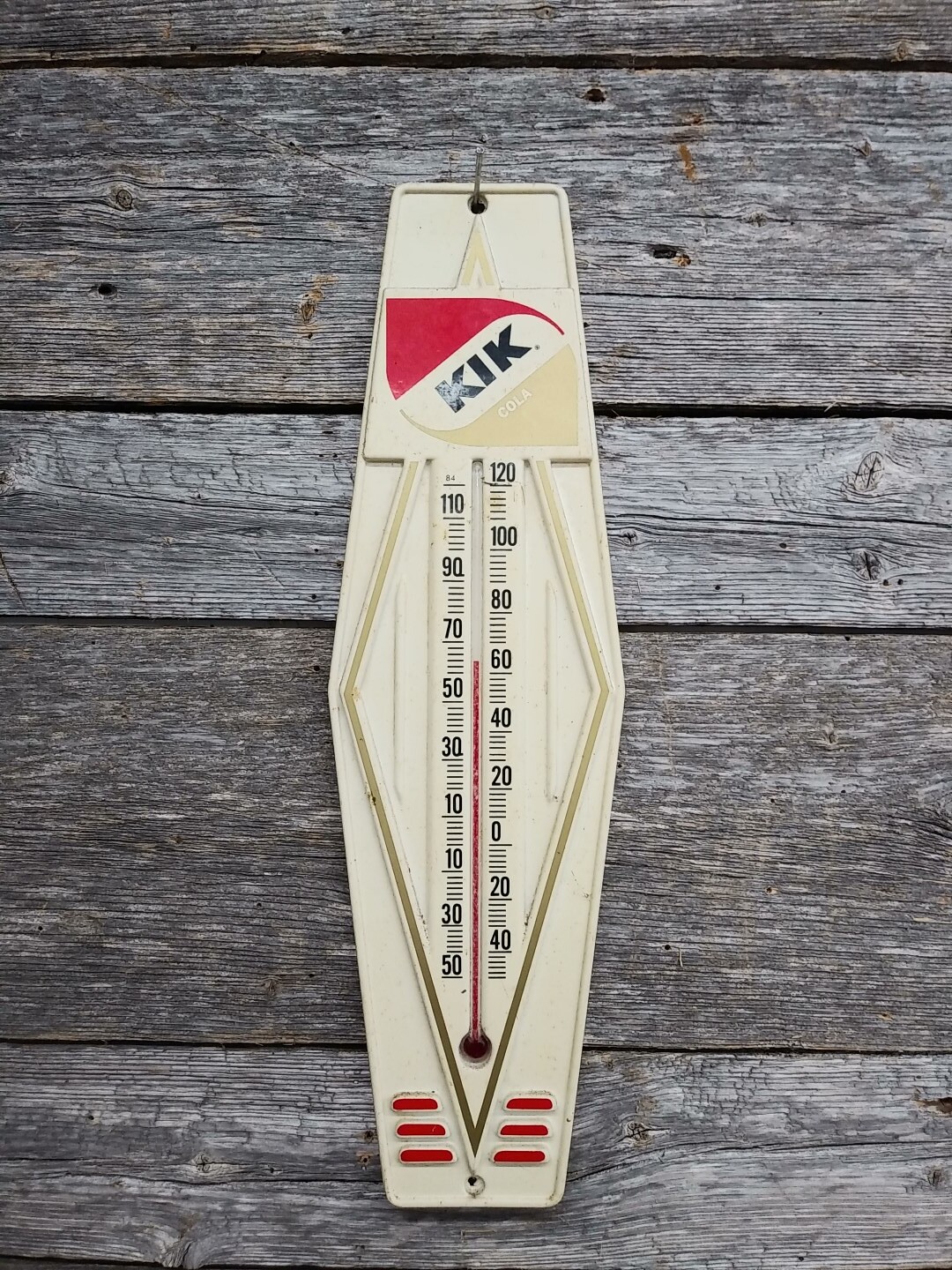The image depicts a highly weathered wooden wall, likely the exterior side of a house, composed of closely set, rough-sawn gray boards. These planks, noticeably rough due to prolonged exposure to the elements, show no signs of paint or stain, highlighting their natural, aged texture. Mounted on this rustic backdrop is a hexagonal plastic thermometer, elongated vertically to appear oblong while still retaining its hexagonal structure. The thermometer, injection molded from tan plastic, features a diamond-shaped inset that frames the actual temperature gauge.

At the top of the thermometer, there's a distinctive logo split into two color sections: red on the upper half and tan on the lower, with the letters "KIK" inscribed in either white or a transparent section of the plastic. The visible thermometer inside uses red-tinged alcohol to measure the temperature. Interestingly, although it initially appears to have dual scales, it has a single Fahrenheit scale that runs from minus 50 to plus 120 degrees, with alternating numbers placed on either side of the scale for visual clarity.

The thermometer hangs securely from the wooden wall by a small, thin brad driven into the wood at an angle, utilizing a hole at the top of the thermometer for support. Additionally, for decorative purposes, there are two stacks of three dashes at the bottom of the plastic casing. A second, unused mounting hole is also present at the bottom.

Overall, the combination of the rugged, unpainted boards and the functional, yet slightly ornate thermometer provide a striking contrast, blending utilitarian design with a touch of rustic charm.